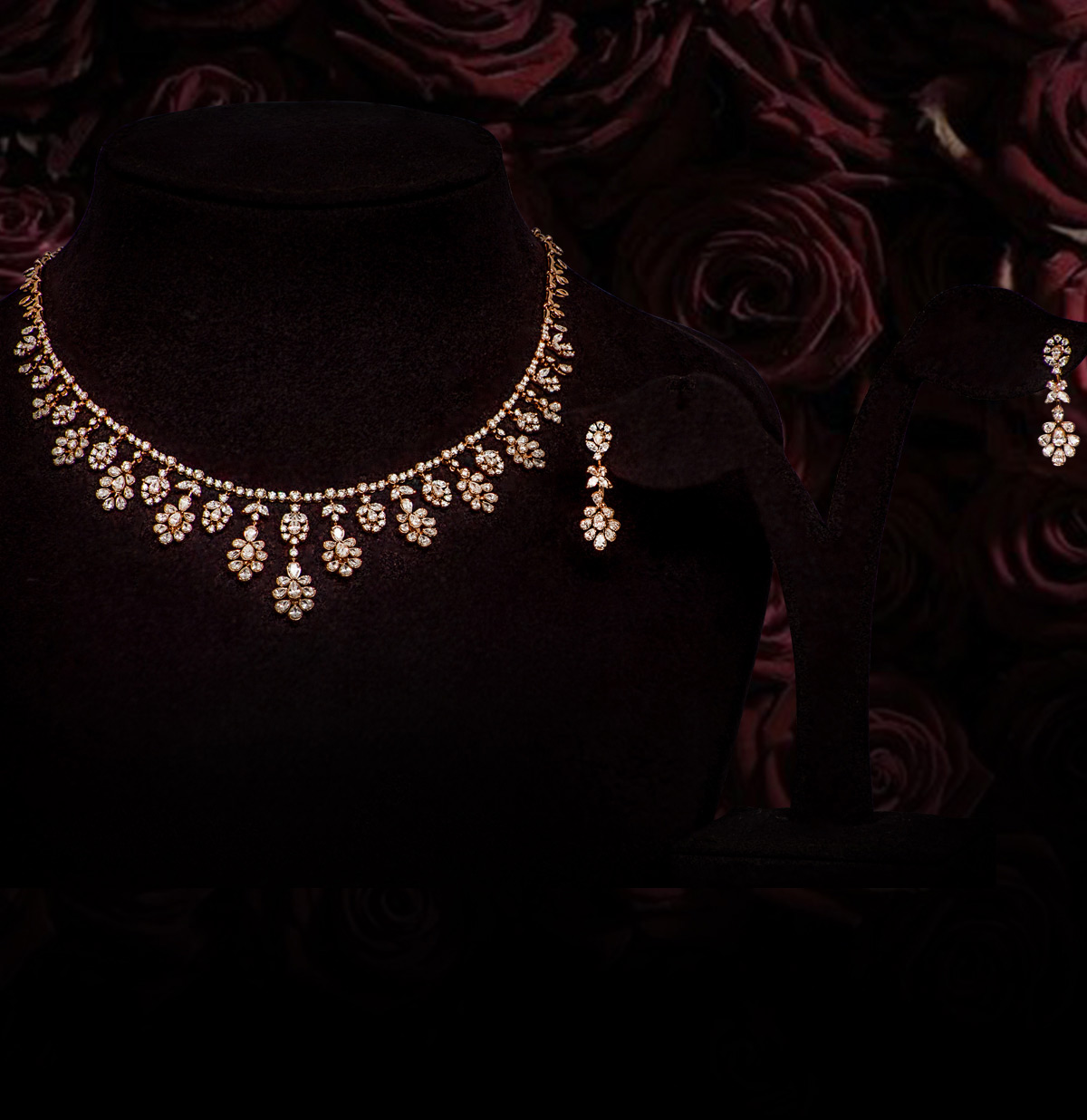In this color photograph, a stark black background sets a dramatic stage, highlighting a monochromatic arrangement of deep wine-red roses that form a collage throughout the upper portion of the image, with some roses extending toward the middle-lower right side. In the foreground, a black mannequin resembling a human torso without the head features a striking silver necklace adorned with diamond flowers, each cascading in a drop-down style with the central diamond hanging the longest. To the right, a black earring holder in the shape of rabbit ears showcases a matching pair of diamond drop earrings, each decorated with intricate flower shapes. This carefully arranged display emphasizes the glittering elegance of the jewelry, which appears to be a meticulously crafted set, potentially from a famous designer or notable collection, though no price or information is provided. The dark, moody lighting of the photograph accentuates the brilliance of the diamonds, allowing the vibrant red roses and the shimmering jewels to stand out in sharp contrast.